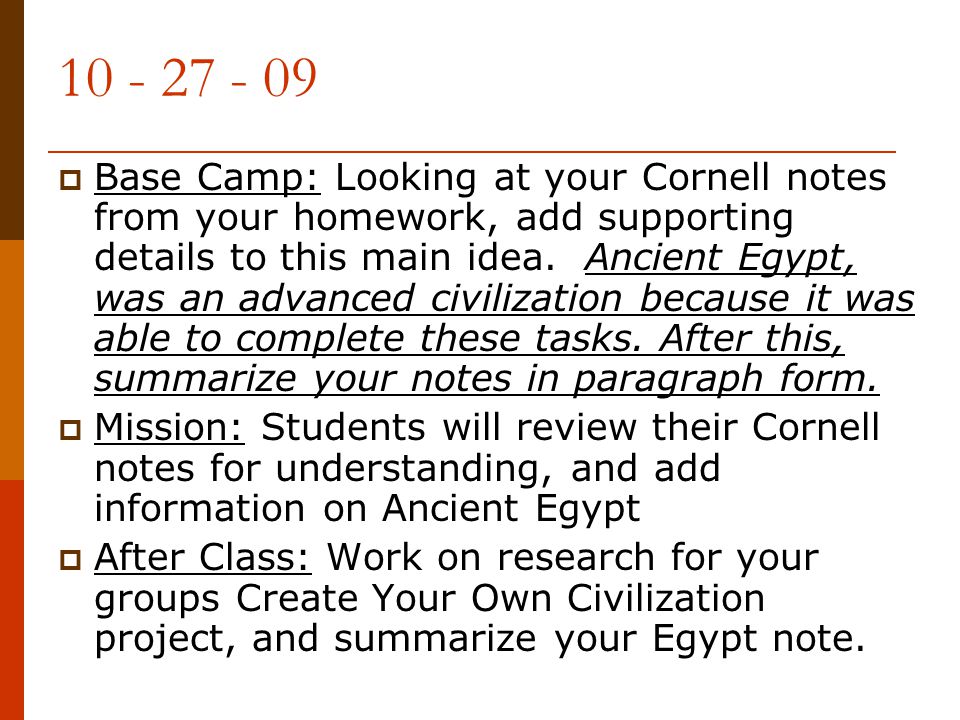The image shows a slide dated 10-27-09, with a tricolor vertical line on the left, transitioning from brown through a lighter brown to red. At the top, a light brown text displays the date "10-27-09," underlined by a thin brown line. Below this line, black text on a white background outlines three main sections, each with an underlined header. 

1. **Base Camp**: Instructions begin with, "Looking at your Cornell notes from your homework, add supporting details to this main idea." The text continues with the underlined and italicized statement, "Ancient Egypt was an advanced civilization because it was able to complete these tasks." The section concludes with, "Summarize your notes in paragraph form."

2. **Mission**: This section states, "Students will review their Cornell notes for understanding and add information on Ancient Egypt."

3. **After Class**: The text advises, "Work on your research for your groups, create your own civilization project, and summarize your Egypt notes."

The combined input provides a comprehensive, detailed description of the image, capturing the essence of each individual's observations.